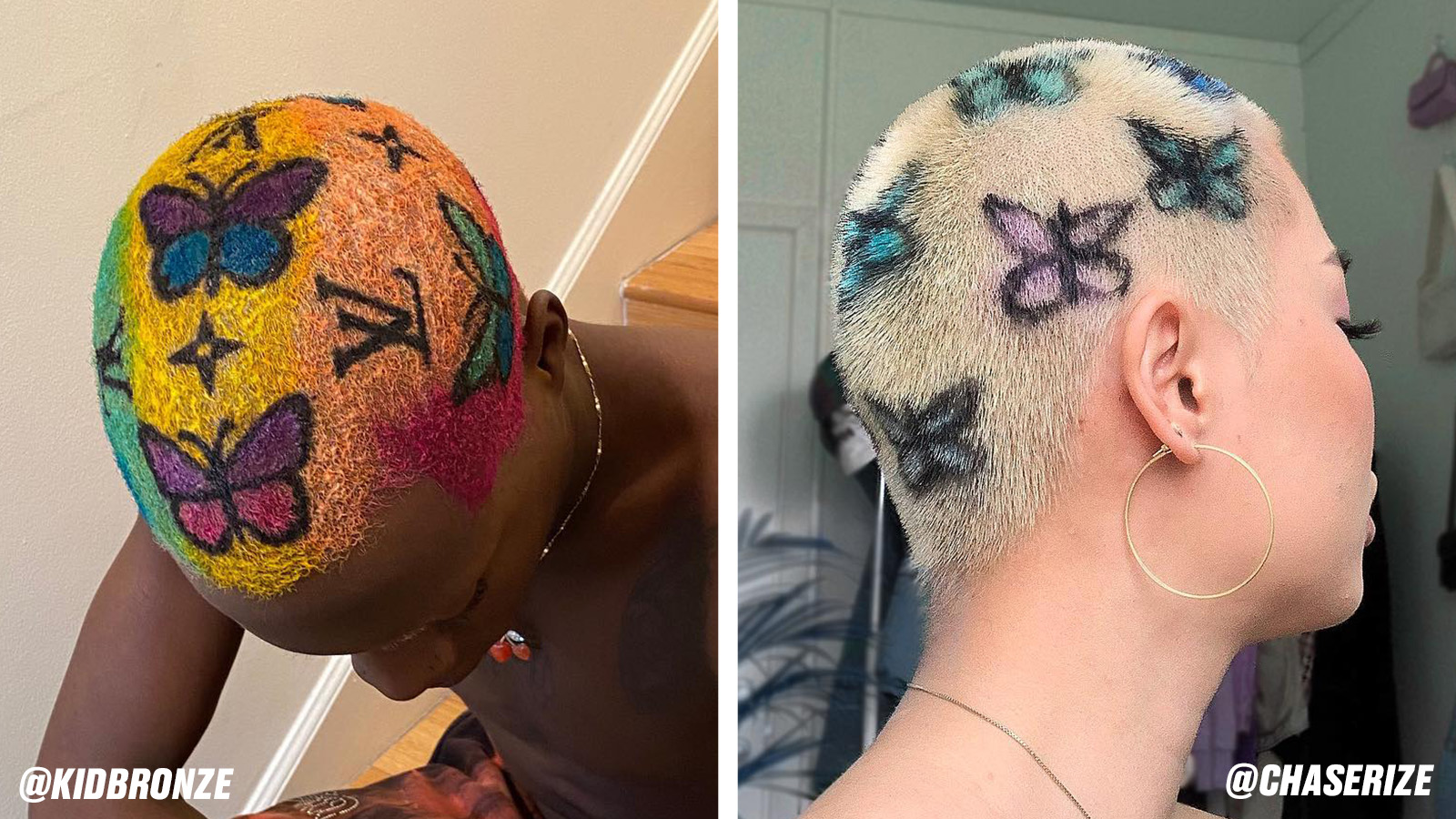This image features two side-by-side photographs showcasing individuals who have had intricate designs dyed onto their hair. On the left, a young black male is seated on a staircase, shirtless, adorned with a thin gold chain around his neck. His hair, shaved very close, is a vibrant canvas of colors: yellow on the top center, pink, green, and red around the sides and back. Detailed illustrations are intricately dyed into his hair, including the Louis Vuitton logo, iconic star shapes, and butterflies with varying wing colors—purple and blue, purple and red, and green and blue. The bottom left corner of his photo bears the handle "Kid Bronze" in all capital letters, adding a signature touch to the design.

On the right, a lighter-skinned African-American woman is captured looking back over her left shoulder to flaunt her hair art. Her hair, also shaved short and dyed a striking blonde, features butterflies airbrushed in soothing shades of teal, blue, and purple. She accessorizes her look with gold hoop earrings and a thin necklace, standing in what appears to be a bedroom with a potted plant and a coat rack visible in the background. The handle "@Chasiris" is elegantly placed in the bottom right corner of her photo.

Together, these two images celebrate the bold and creative expression of hair art, capturing the detailed and colorful designs sported by both individuals.